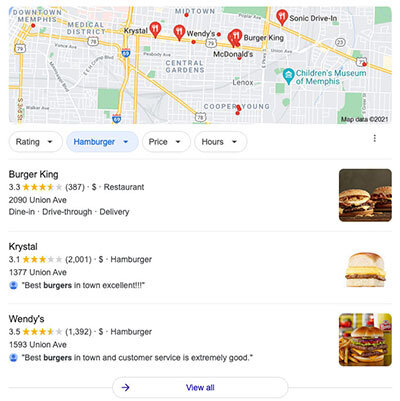The image displays a Google Maps search result page showcasing a detailed map with several red pin markers indicating fast food restaurant locations in various areas around downtown Memphis, including the Medical District, Midtown, Central Gardens, Cooper-Young, and near the Children's Museum of Memphis. At the top of the page is a street scene, giving a visual context to the map.

Below the map, there are listings for specific fast food restaurants, including their ratings, reviews, pricing, categories, addresses, and services. 

1. **Burger King**: 
   - Rating: 3.3 stars 
   - Reviews: 387 
   - Price: $ 
   - Category: Restaurant 
   - Address: 2090 Union Avenue 
   - Services: Dine-In, Drive-Thru, Delivery

2. **Krystal**:
   - Rating: 3.1 stars 
   - Reviews: 2001 
   - Price: $ 
   - Category: Hamburger 
   - Address: 1377 Union Avenue
   - Highlighted review: "Best burgers in town, excellent."

3. **Wendy’s**:
   - Rating: 3.5 stars 
   - Reviews: 1392 
   - Price: $